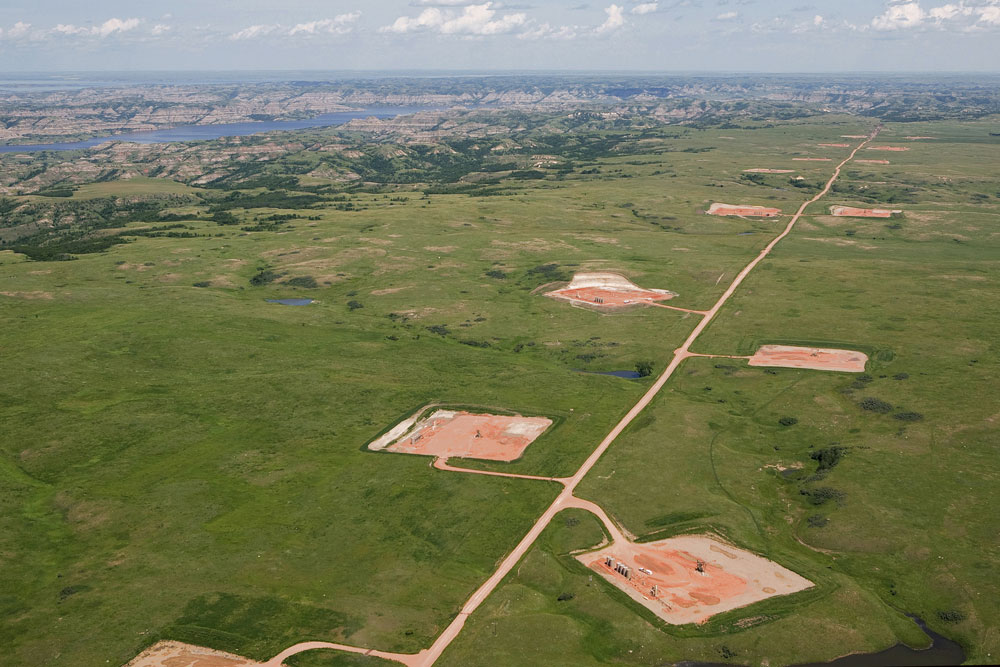This aerial photograph, likely taken from a drone or helicopter, showcases a vast countryside dominated by a long, light-brown gravel road that stretches from the bottom middle of the image, winding upwards and slightly to the right. Branching off from this main gravel road are numerous short gravel drives, leading to square plots of similarly colored brown land, suggesting early-stage construction sites. Surrounding these plots and drives is an extensive expanse of green grassland, mostly flat and devoid of trees, giving the landscape a serene, pastoral appearance.

In the upper left corner of the image, there is a noticeable cluster of trees that forms a small wooded area, adjacent to what appears to be a developed region characterized by brown hues and speckled with potential buildings. Just below this cluster, a body of water extends out and to the right, adding a contrasting element to the scene. Beyond the end of the main gravel road, in the upper right-hand corner, a mix of green and brown terrain is visible, though indistinct due to distance. The top of the image is adorned with white clouds scattered across a grayish sky, completing this comprehensive view of the landscape.